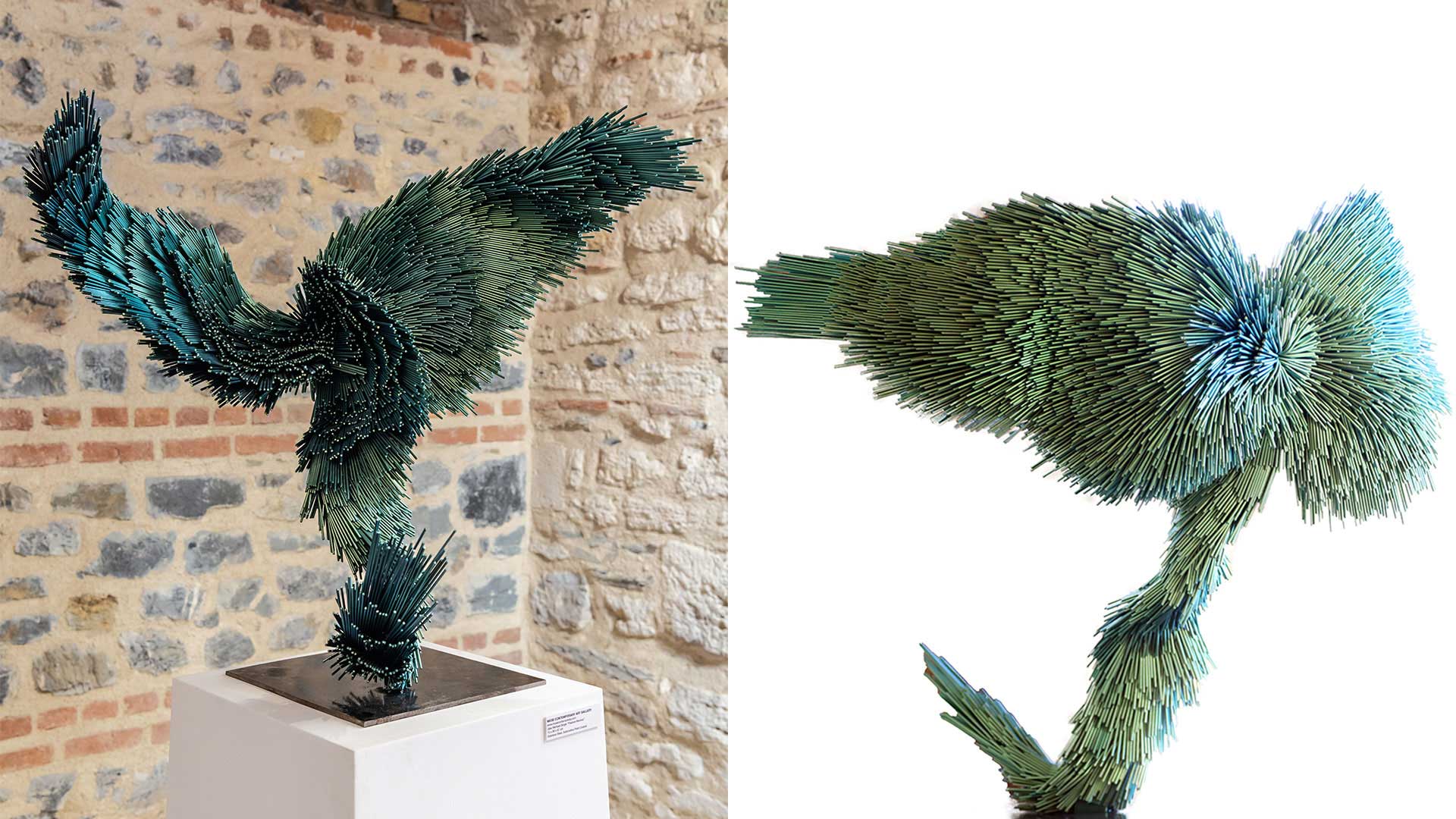The image features two views of the same intricate sculpture. The left-hand photo captures the sculpture positioned on a black bronze base atop a white pedestal, which includes a small, unreadable museum sign. The background in this image is a distinctive brick and stone wall with visible grout, incorporating pinkish-red and gray bricks. The right-hand photo presents the sculpture against a simple white background, highlighting its detailed craftsmanship from a different angle.

The sculpture itself resembles an eagle with outstretched wings, meticulously crafted from numerous blue-green rods. These rods give the appearance of feathers or pine needles, forging a three-dimensional pattern. The wings are asymmetrical and curve in varied directions, adding to the dynamic form of the piece. The juxtaposition of the sculpture against both the textured brick wall and the plain white background helps to emphasize its intricate detail and artistic complexity.